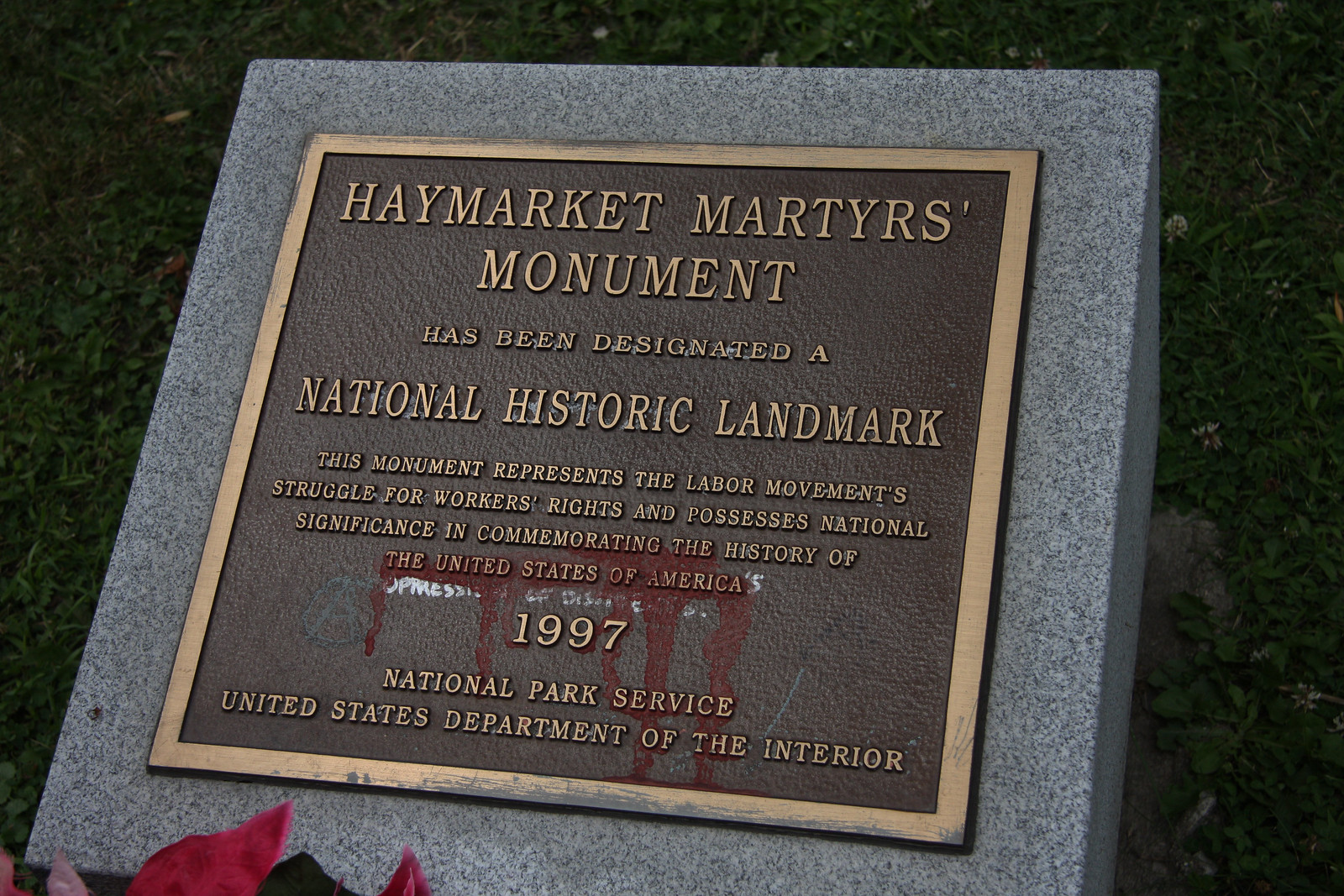The photograph depicts a prominent stone monument set in a field of green grass, scattered with fallen leaves and flowers. The monument is made of a gray, granite-like material, with a plaque that features a brown background and gold-colored text and border. The plaque reads, "Haymarket Martyrs Monument has been designated a National Historic Landmark. This monument represents the labor movement's struggle for workers' rights and possesses national significance in commemorating the history of the United States of America." Below this inscription, in a smaller font, is the year "1997" followed by "National Park Service United States Department of the Interior." All the text on the plaque is in capital letters and rendered in a serif font. Additionally, there is a notable detail in the lower left corner of the image where red petals or possibly a red liquid, resembling blood, are visible on the grass surrounding the monument.